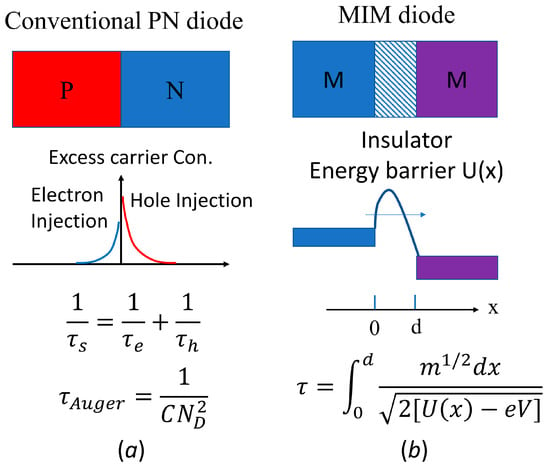This detailed image is a color-infographic depicting technical information about two types of diodes: a conventional PN diode and a MIM diode. The infographic is landscape-oriented, with the two diagrams placed side-by-side in portrait orientation.

On the left, labeled "A," is a conventional PN diode. This section includes a divided rectangle with the left side in red (marked "P") and the right side in blue (marked "N"). A diagram within this section shows "Excess Carrier CON" and delineates "Electron Injection" with a blue line and "Hole Injection" with a red line. Below this diagram, various mathematical equations are provided, including \( \frac{1}{TS} = \frac{1}{TE} + \frac{1}{TN} \) and \( \tau_{\text{auger}} = \frac{1}{CN} 2 \over D \).

On the right, labeled "B," is the MIM diode. This section features a rectangle divided into three parts: a large blue area on the left labeled "M," a central shaded area representing the insulator energy barrier ("U(x)"), and a purple area on the right also labeled "M." A diagonal line marks the insulator energy barrier, with a blue line extending to the top left of the purple section and a curved line arching towards the right, indicating energy transfer. Key equations in this section include \( T = \frac{D}{O} \) and \(\frac{M \frac{1}{2}}{\frac{1}{2}} \cdot \frac{Dx}{\sqrt{2}} [U(x) - Ev] \).

Both diagrams are accompanied by additional line art graphs and scientific notations that provide a deeper insight into the electrical properties and behaviors of the diodes being explained.